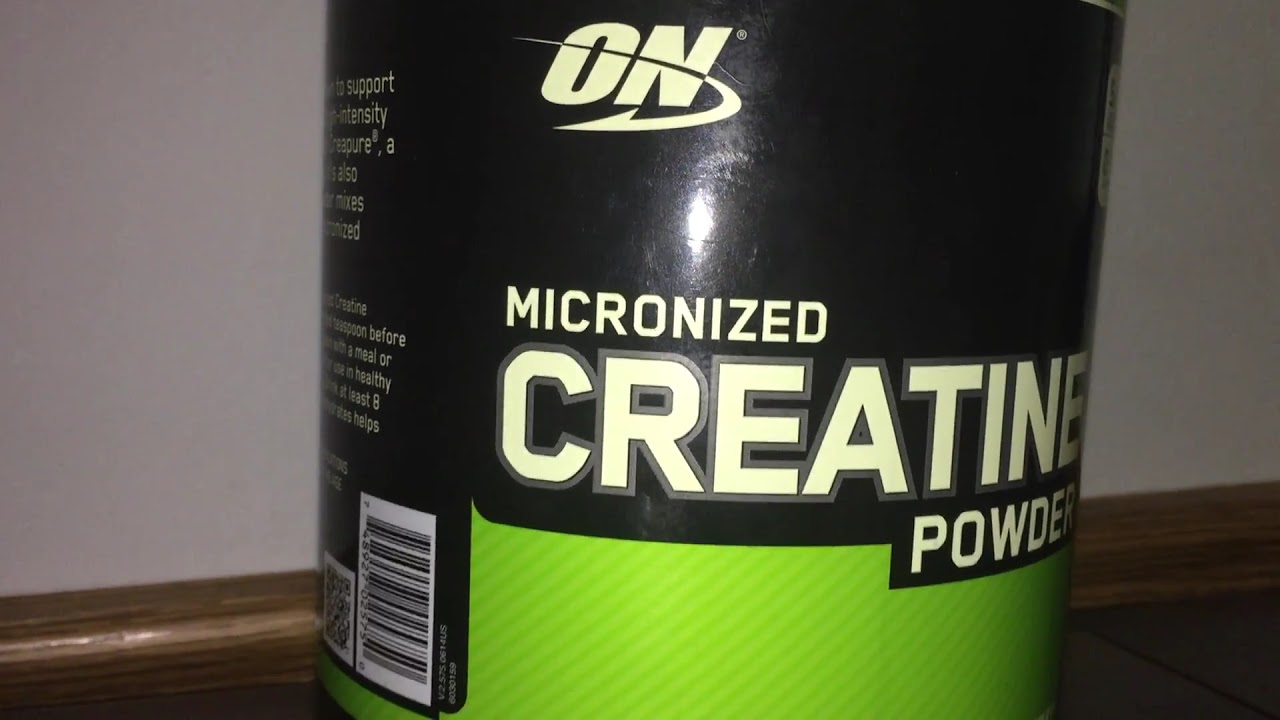In this detailed color photograph, the central focus is a large tub of creatine powder, prominently positioned in the center of the image. The bottle appears to be placed directly on a tile floor against a backdrop of a white wall with visible crown molding, suggesting an indoor setting, possibly someone's kitchen or bedroom. The bottle, in decent condition, features a distinct black label with the bold, white text "Micronized Creatine Powder," accompanied by a gray shadow effect. The upper section of the label showcases the "ON" logo in italicized white lettering with a decorative arrow swirl. A bright green band wraps around the lower portion of the bottle, along with a visible UPC code and partially legible descriptions hinting at the product’s benefits, including words such as "support," "intensity," and "healthy." The photograph's landscape orientation frames the bottle to occupy the entire height of the image and about two-thirds of its width, emphasizing the label's clarity and details through a zoomed-in perspective.